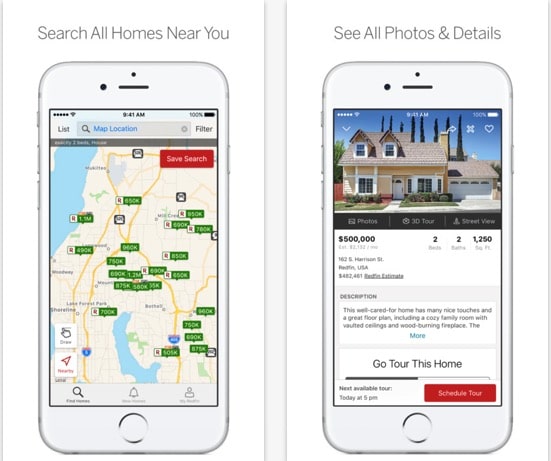The image consists of two separate smartphone screenshots placed side by side vertically. Both smartphones are a light gray or white color, each bordered by vertical light gray lines. 

On the left side, the caption above the phone reads, "Search all homes near you." The smartphone screen displays a map with various green boxes marked with prices, indicating the cost of homes in different areas. Additional features on this screen include a "Nearby" button and a red "Save Search" button. The address bar at the top reads "Map Location."

The right side of the image is captioned, "See all photos and details." The smartphone on this side shows a photograph of a two-story ranch-style house with a garage at the top of the screen. Below the photo, the house is listed at $500,000 and has a size of 1,250 square feet. The location is noted as East Harrison Street. Beneath this, there is a descriptive text box, followed by a prompt that reads, "Go tour this home" and a red "Schedule Tour" button.

These elements together provide a comprehensive view of the functionalities available in a real estate app, showcasing both map-based searches and detailed property listings with photos and touring options.